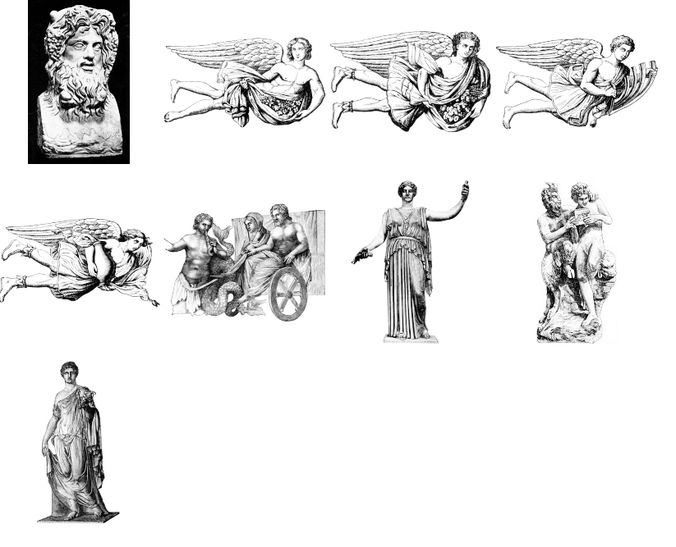The set comprises nine grayscale images arranged in three rows against a solid white background, each depicting sculptures, busts, and illustrations reminiscent of ancient Greek or Roman art. The top row starts with a vertical rectangular image featuring a sculpted bust of a man with a full, lion-like beard and long hair on a black background. To its right, three images display male angelic figures in classic style: the first angel appears inactive or reclining; the second is flying; and the third holds a woodwind instrument, possibly a calliope, while flying. All angels are dressed in togas, with some carrying fruit in their sashes.

In the middle row, the first image shows another angel, with its gender indistinguishable, seemingly flying or tilted. The next image depicts a small scene featuring a shirtless man handling a wheel, another individual, and a large serpent, suggesting an animated discussion. Following this, a regal male figure stands with one arm raised, draped in a long sash with possible laurels behind his ears. This is succeeded by an illustration of a satyr—half-goat, half-man—tempting a seemingly amused, potentially nude woman.

The lone image in the bottom row presents a statue of a man dressed in a toga, standing prominently with one shoulder exposed and exuding an emperor-like demeanor. This comprehensive collection highlights the artistic richness and classical heritage of Greco-Roman civilization.